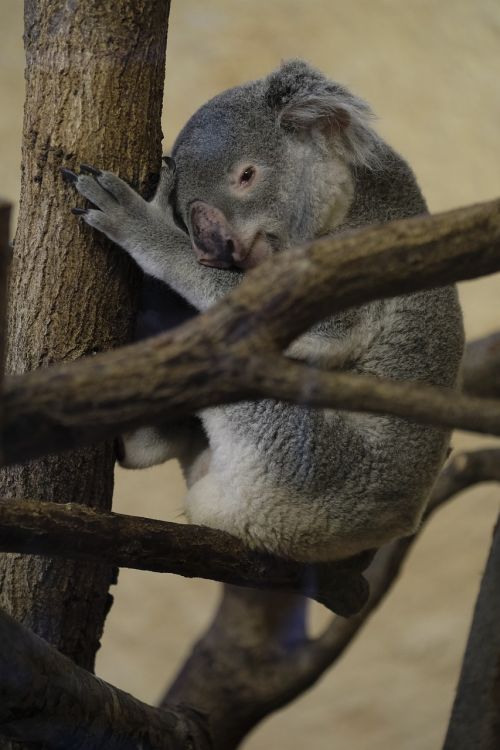A gray koala bear is perched on a bare, brown tree branch, which seems to be more of a zoo climbing structure than a real tree due to the lack of foliage. The koala's soft gray fur and distinct long fur from around its ears are clearly visible as it looks directly at the camera. Its dark gray, almost black claws are gripping the main trunk with its nose resting on its left paw. The koala's facial features show a lighter patterned gray around its eyes and a cream-gray coloring below its ears. The background is blurred and consists of neutral tan and stony colors, creating an indistinct setting that suggests either an outdoor or a zoo environment. The overall image emphasizes the koala's calm and centered presence amid the muted tones of its surroundings.